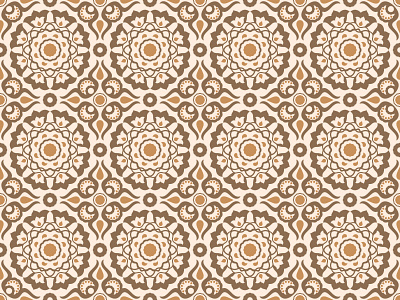The image depicts a detailed and ornate pattern that could be suitable for wallpaper or tile design. The pattern has a neutral palette dominated by browns, golds, and light beiges, all set against an off-white background. There are three rows of large circles, each consisting of flower-like shapes with light brown centers. Surrounding each of these circles are smaller floral designs that fill the spaces between the larger circles, creating a geometric and mosaic-like appearance. The spaces between the circles form squares and diamond shapes composed of intricate floral and triangular components, giving the pattern a busy and richly decorative look.